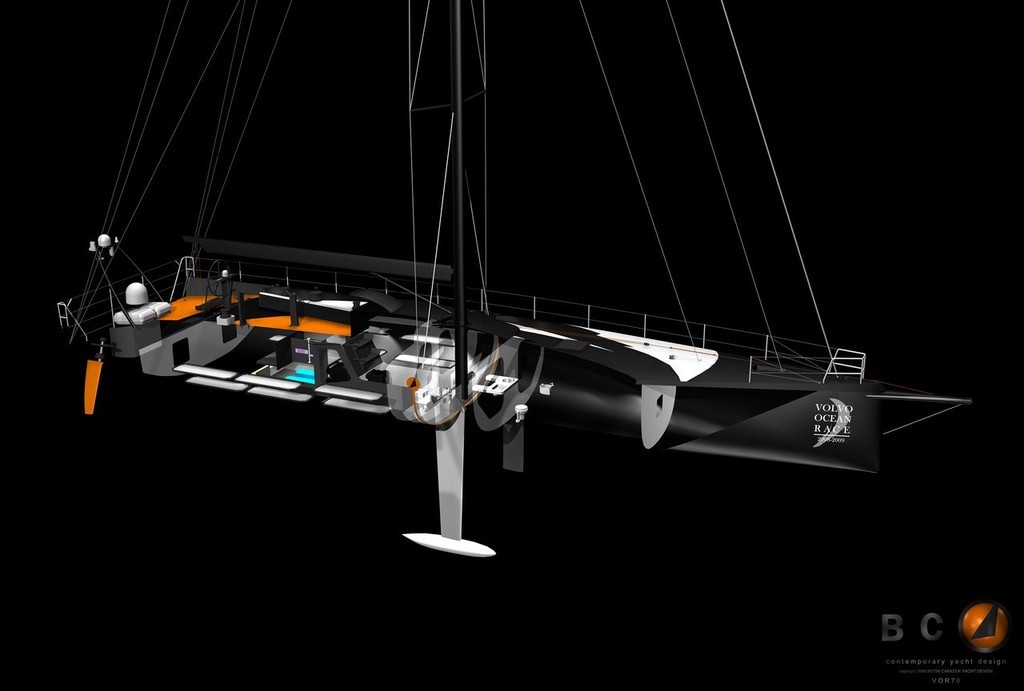The image is a digitally crafted depiction of a sea vessel, possibly a boat or a submarine, horizontally aligned against a solid black background. The vessel is predominantly black and silver, featuring a transparent structure that reveals multiple compartments inside. It spans from the left, where it appears to have a steel guardrail, to the right. The vessel's frontal, right side has text that reads "Volvo Ocean Race." At the vessel's center, a vertical black rod extends upward, resembling where a sail might be. Surrounding this rod are silver wires stretching from top to bottom. The top levels of the vessel have orange flooring, and a small orange section is visible near the back. The vessel features silver bars and a possible propeller-like structure at the bottom. A notable detail within the image is a logo in the lower right corner, characterized by gray letters "B" and "C," and an orange shaded "O" with a black triangle inside it.